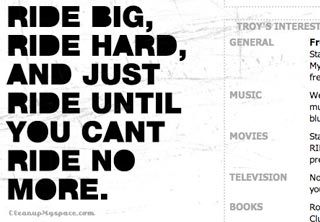The image features a small white background with a subtle pattern and bold black text on the left side that reads, "Ride Big, Ride Hard, and Just Ride Until You Can't Ride No More," spread across seven left-aligned lines. Due to the boldness of the letters, enclosed spaces such as those in 'B' and 'D' are filled in with black. On the right side, there is gray text that reads "Troy's Interest" followed by categories "General, Music, Movies, Television, and Books." These categories extend into columns that are partially cut off, making the words on the far right indistinguishable. At the bottom left of the image, there is a faint, difficult-to-read URL in gray font.